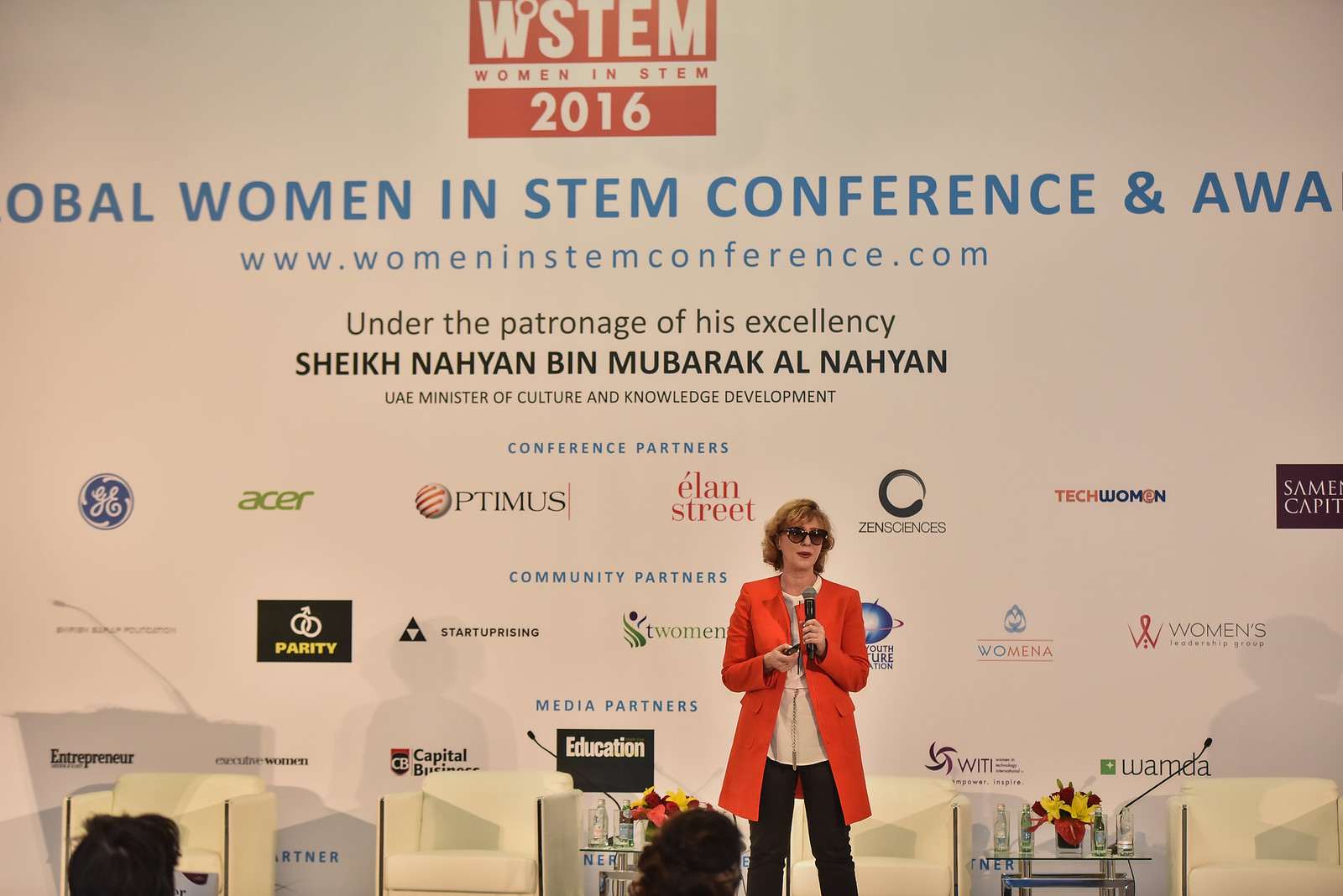In this detailed photograph, a woman in her 40s stands on stage at the 2016 WSTEM (Women in STEM) conference. She has dirty blonde hair cut short, just above her shoulders, and is sporting sunglasses. Her outfit includes a striking red trench coat over a white shirt, paired with black pants. In her right hand, she holds a microphone close to her mouth, and in her left, she holds a remote control, likely for a projector. Facing the audience, she's engaged in delivering her speech. 

The backdrop features significant text, starting from the top, in bold red, "WSTEM Women in STEM 2016." Below, in blue text, it reads "Global Women in STEM Conference and Awards." The white and red text contrasts against the large white background. Further down, the website "www.womeninstemconference.com" is prominently displayed. Beneath that, text in black reads, "Under the patronage of His Excellency Sheikh Nahyan Bin Mubarak Al Nahyan, UAE Minister of Culture and Knowledge Development."

A series of logos for conference partners are visible, including notable names like GE in blue, Acer in green, Optimus in black and red, Elan Street in red, Zen Sciences in black, Tech Women in orange and blue, and several others. The stage is furnished with four small chairs and two glass tables adorned with floral decorations and equipped with boom microphones. The shadowy outlines of two audience members can be seen at the bottom of the frame, attentively listening to the speaker. This vivid scene captures a moment of shared knowledge and celebration of women's contributions to the STEM fields.